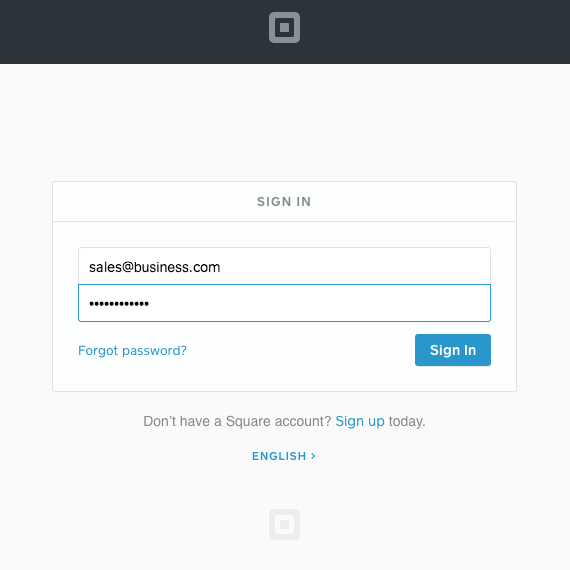**Caption:**

A screenshot of the Square login page is displayed. The background of the web page is a very faint gray, encompassing the entire rectangular screen. At the top, a wide black header spans across the page, centered with a distinct icon. This icon consists of a larger gray square enclosing a smaller black square, which further encases another gray square.

Below this header, the main section of the page features a prominent white rectangular box, outlined in pale gray and occupying about one-third to one-half of the screen's width. At the top of this white box, "SIGN IN" is written in gray uppercase letters, followed by a faint gray line underneath it.

The login section within this white box is divided into two halves. The upper half contains the username field, pre-filled with "sales@business.com" in black text. The lower half, highlighted in bright blue, is the password field, obscured by dots to represent hidden characters. Below the password field, "Forgot password?" is displayed in bright blue text.

To the right of the password input, a bright blue button with white text reads "SIGN IN". Beneath this white box, a message in gray text states, "Don't have a Square account?". The phrase "Sign up today" follows, with "Sign up" in bright blue.

Finally, at the bottom of the page, the word "ENGLISH" appears in bright blue uppercase letters, accompanied by a forward arrow symbol.